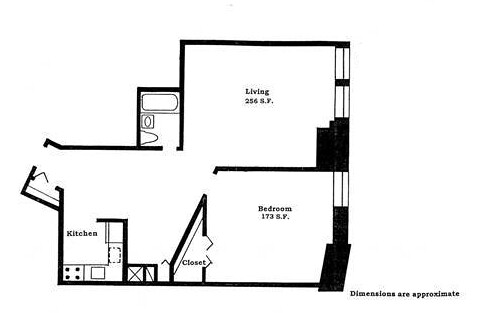This image depicts a detailed floor plan with approximate dimensions indicated in black font. The layout includes several rooms clearly labeled with their respective sizes. 

To the left, there is a living room marked "Living - 256 SF," showcasing an expansive main area. Below the living room, the bedroom is labeled "Bedroom - 173 SF," featuring a walk-in closet indicated by an opening. 

Adjacent to the bedroom is the kitchen, illustrated with a drawing of a stove and a kitchen sink, providing a clear sense of the workspace available. 

Additionally, the floor plan includes a bathroom, identifiable by a sketch of a bathtub, a small kitchen sink, and a door opening. This comprehensive blueprint offers a clear understanding of the spatial arrangement and primary features of each room.